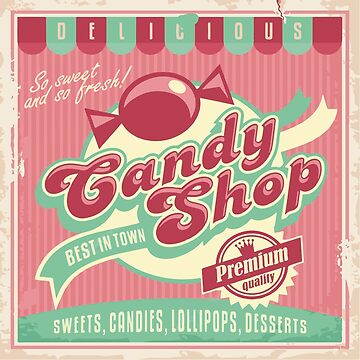The image is a vibrant advertisement for a store called the Candy Shop, characterized by its striking pink and mint green tones. At the top of the sign, the word "Delicious" is displayed prominently in a red and Tiffany blue pattern, with each letter set in individual squares. Beneath this, the catchy slogan "So sweet and so fresh!" is written in white. A stylized drawing of a pink wrapped candy accents the sign, which is encircled by the store's name, "Candy Shop," written in a beautiful pink font. Below the store name, the tagline "Best in town" and a crowned seal proclaiming "Premium Quality" are featured, emphasizing the high standards of their products. The bottom section lists the variety of offerings available: "Sweets, Candies, Lollipops, Desserts," all written in white on a mint green background with a deliberate aging effect. The entire sign is bordered in white, giving it a vintage, worn look that adds to its charm.